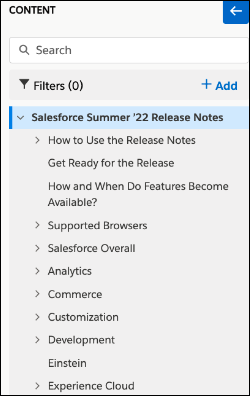This screenshot, possibly taken on either a mobile device or a PC, showcases a Salesforce interface. The header at the top clearly indicates "Content," accompanied by a search bar featuring a magnifying glass icon. Below the header, there are several sections of text. It begins with "Salesforce Summer '22 Release Notes," followed by subsections labeled "How to Use Release Notes," "Get Ready for Release," "How and When Do Features Become Available," and "Supported Browsers," with an adjacent right-facing arrow indicating a dropdown menu.

Additional sections listed include "Salesforce Overall," "Analytics," "Commerce," "Customization," "Development," "Einstein," and "Experience Cloud." This layout suggests that the document is a comprehensive guide or reference for Salesforce employees, likely intended for internal use to provide detailed information on the various aspects and updates of the Salesforce platform. The inclusion of multiple sections and subsections supports its purpose as a thorough reference resource, aimed at answering questions and providing guidance on the platform's features and capabilities.